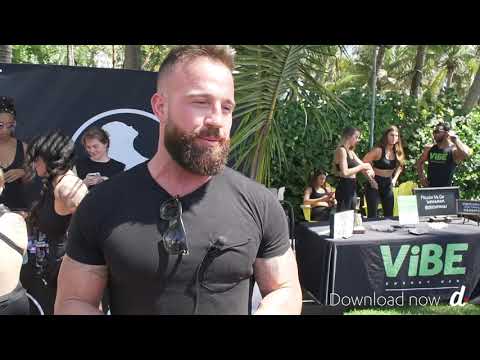The image features a well-muscled Caucasian man in his 30s with short brown hair and a long brown beard, standing at the center. He is wearing a gray t-shirt with sunglasses hanging from the neckline. He seems to be mid-conversation, perhaps in an interview, suggested by a possible mic in his shirt pocket. In the background, on the right side, there is a table draped in a cloth with the word "VIBE" in turquoise letters and the phrase "Download Now" beneath it. On and around the table, several people are engaged, including a black man in a tank top featuring the word "VIBE" and women in sports bras and sweatpants, some checking their phones or watches. The scene appears lively with more individuals in casual wear conversing in the backdrop, four of whom are on the left side talking amongst themselves. The setting hints at a tropical location with visible palm trees and greenery. The photo is bordered by black bars on the top and bottom, and a watermark reading "Download Now D" is visible below.